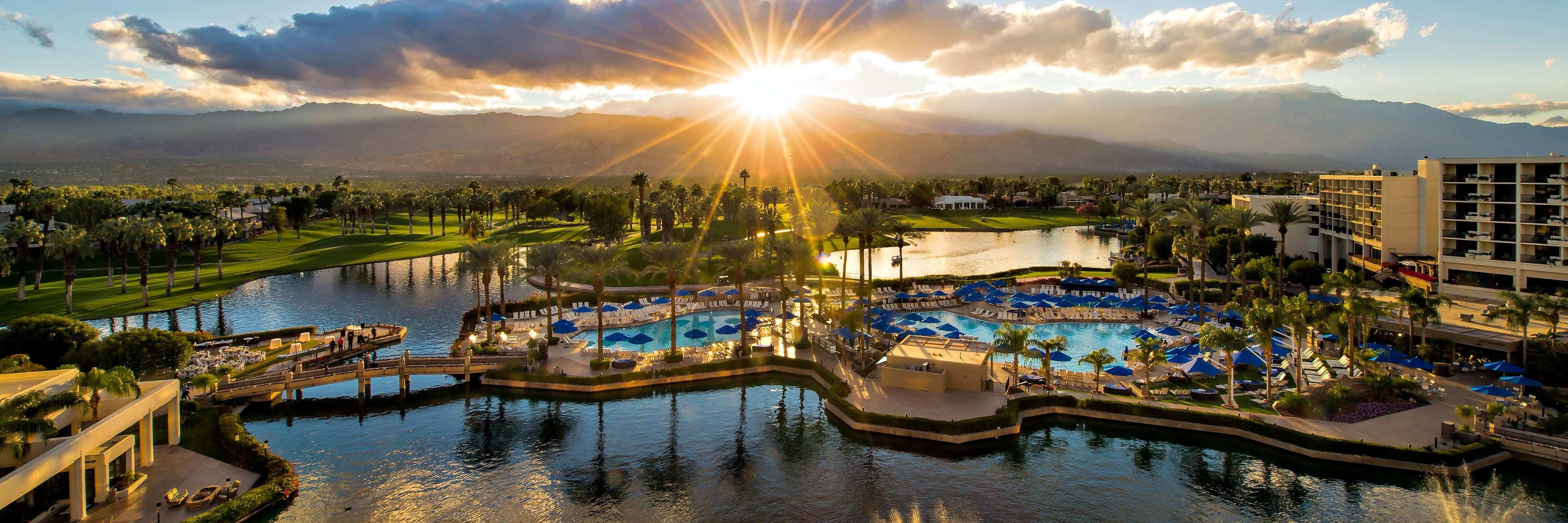This panoramic overhead photograph captures a luxurious resort at sunset, bathed in a bright and radiant sky with sun rays piercing through scattered clouds. Majestic mountains span the background as the sun sets behind them, casting a golden reflection upon the clouds. The resort is surrounded by lush greenery, manicured grass, and tall palm trees, enhancing its tropical allure. Central to the image is a pristine blue swimming pool, bordered by blue umbrellas and sun loungers, seemingly floating on an expansive lake. Intricate walkways and bridges stretch over the water, connecting various parts of the resort. On either side of the image, white and black hotel buildings frame the scene, with visible rooms and possibly a parking ramp on the right, embodying the epitome of luxury and relaxation against the breathtaking natural backdrop.